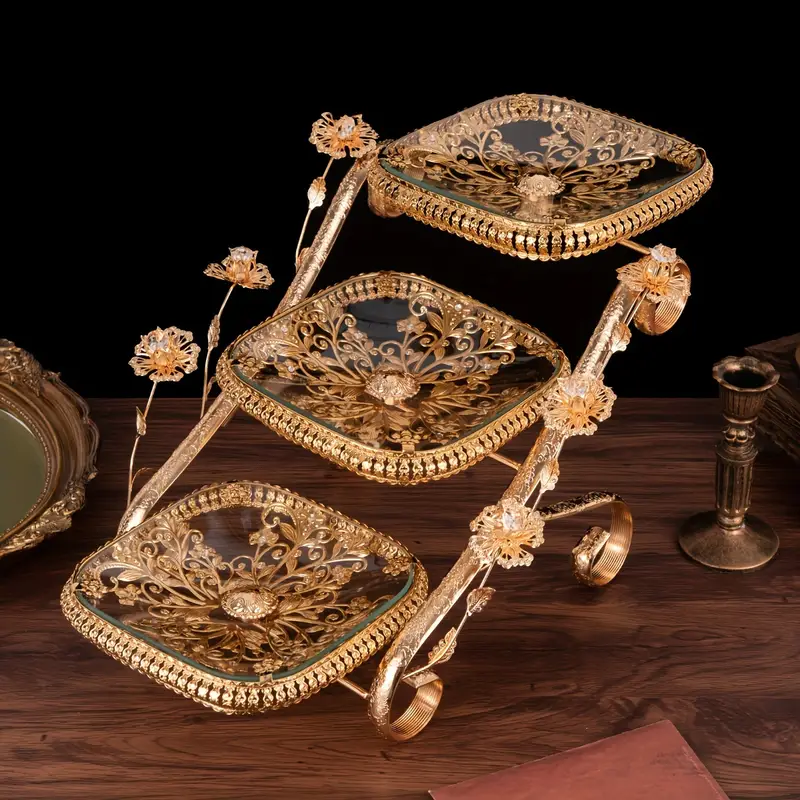In this photograph, set against a black and dark background, a richly detailed, dark wood table is adorned with several ornate objects. Dominating the scene, centrally positioned, is an elaborate three-tiered tray with golden edges. The tray, which stands empty, has flat circular sections embellished with gold floral patterns and connected by gilded elements that give it a bejeweled appearance. These sections appear to have a reflective, glass-like surface, and delicate flower stems project outward along the edges. On the right side of the image, towards the middle, stands a brass candlestick, modestly reaching a couple inches high, sans candle. To the left of the tiered tray, there is a flat, rectangular mirrored tray with a gold frame that can serve as a decorative display base. In the foreground, a brown napkin or piece of paper rests unobtrusively. The overall composition of the image highlights the opulence of the gold accents and the intricate, floral designs against the dark base, creating a visually luxurious scene.